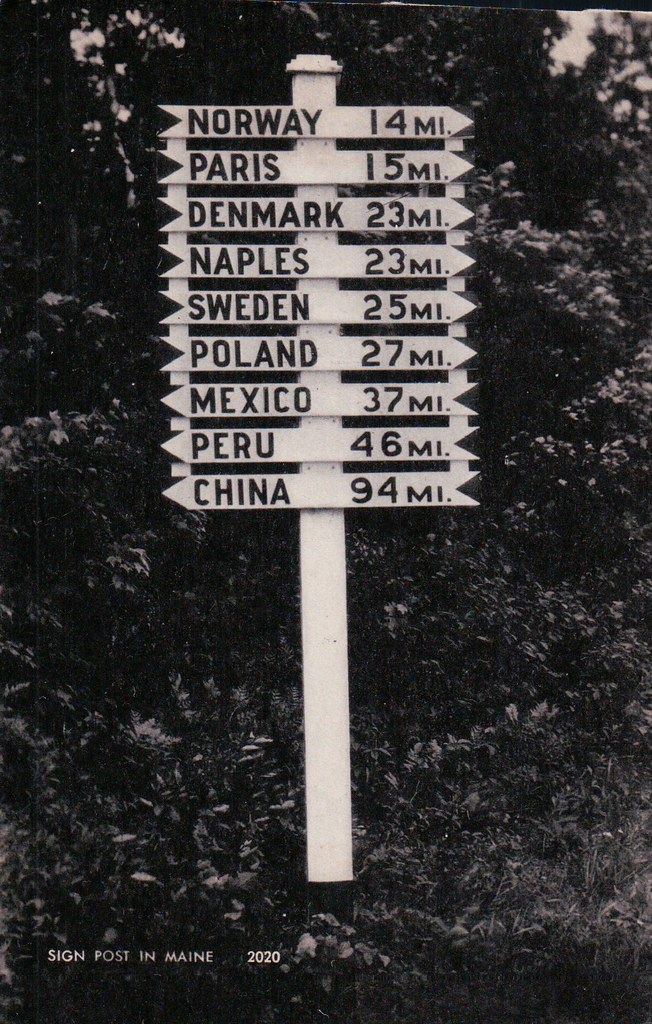This black-and-white photograph, which appears to be quite old, features a white wooden post prominently positioned in the center of the image. The post is adorned with nine directional arrow signs, each pointing toward various distant locations. The signs, all crafted in a uniform long arrow shape, are layered one above the other. 

At the top of the post, an arrow points right with "NORWAY" inscribed in bold black capital letters, indicating a distance of 14 miles. The subsequent arrows follow a similar format, guiding towards different destinations with corresponding distances: "PARIS" at 15 miles, "DENMARK" at 23 miles, "NAPLES" at 23 miles, "SWEDEN" at 25 miles, and "POLAND" at 27 miles, all pointing to the right.

Three arrows point to the left: "MEXICO" at 37 miles, "PERU" at 46 miles, and "CHINA" at a considerable 94 miles. These signs collectively create a vivid tapestry of far-flung locales, hinting at a whimsical or perhaps even an artistic representation rather than actual geographic proximity.

Behind the post, a dense backdrop of lush bushes or tree leaves creates a leafy wall that contrasts with the stark white post and its arrows. At the bottom left of the image, in white capital sans-serif letters, the photograph is labeled: "SIGN POST IN MAINE, 2020." This detail anchors the image in a specific, although somewhat incongruous, time and place, adding to its intriguing nature.